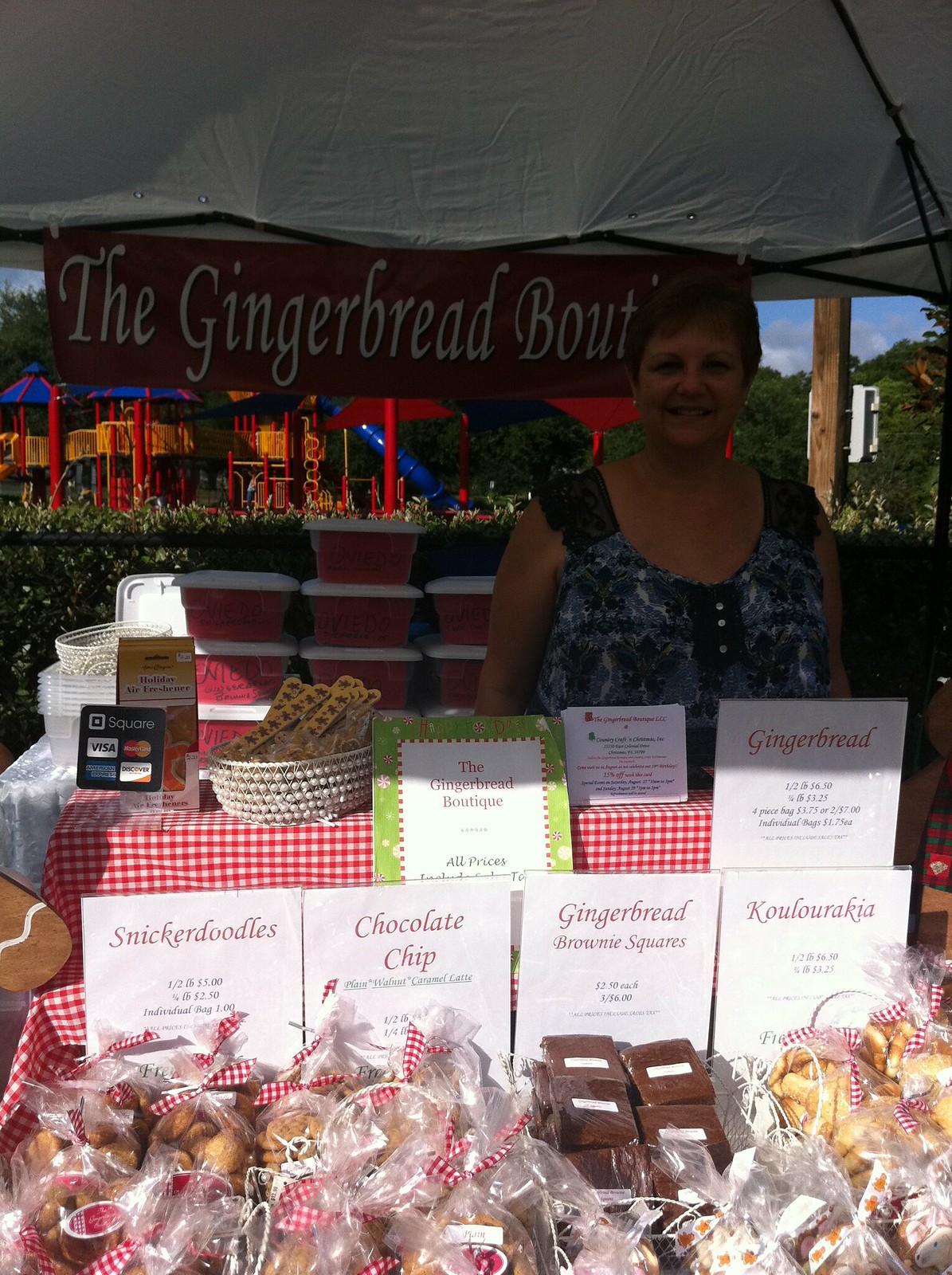The image depicts a lively booth at a farmer's market, set up under a spacious canvas tent resembling a mini pavilion. A sign with partially obscured white text reads "The Gingerbread Boutique" behind a woman with short brown hair, smiling warmly at the camera. She stands in front of a table draped with a red and white gingham tablecloth, displaying a variety of neatly packaged treats. Each treat is showcased in a basket and tied with red and white checkered ribbons. The baskets contain snickerdoodles, chocolate chip cookies, gingerbread brownie squares, and Koulourakia. Various plastic containers and stands with white labels surround her, adding to the organized and inviting setup. In the background, a children's playscape with blue and red elements, wooden rails, grass, trees, and a partly visible sky contribute to the charming outdoor setting. Signs at the front mention payment options like Visa and Mastercard, making the market stand both welcoming and convenient for customers.